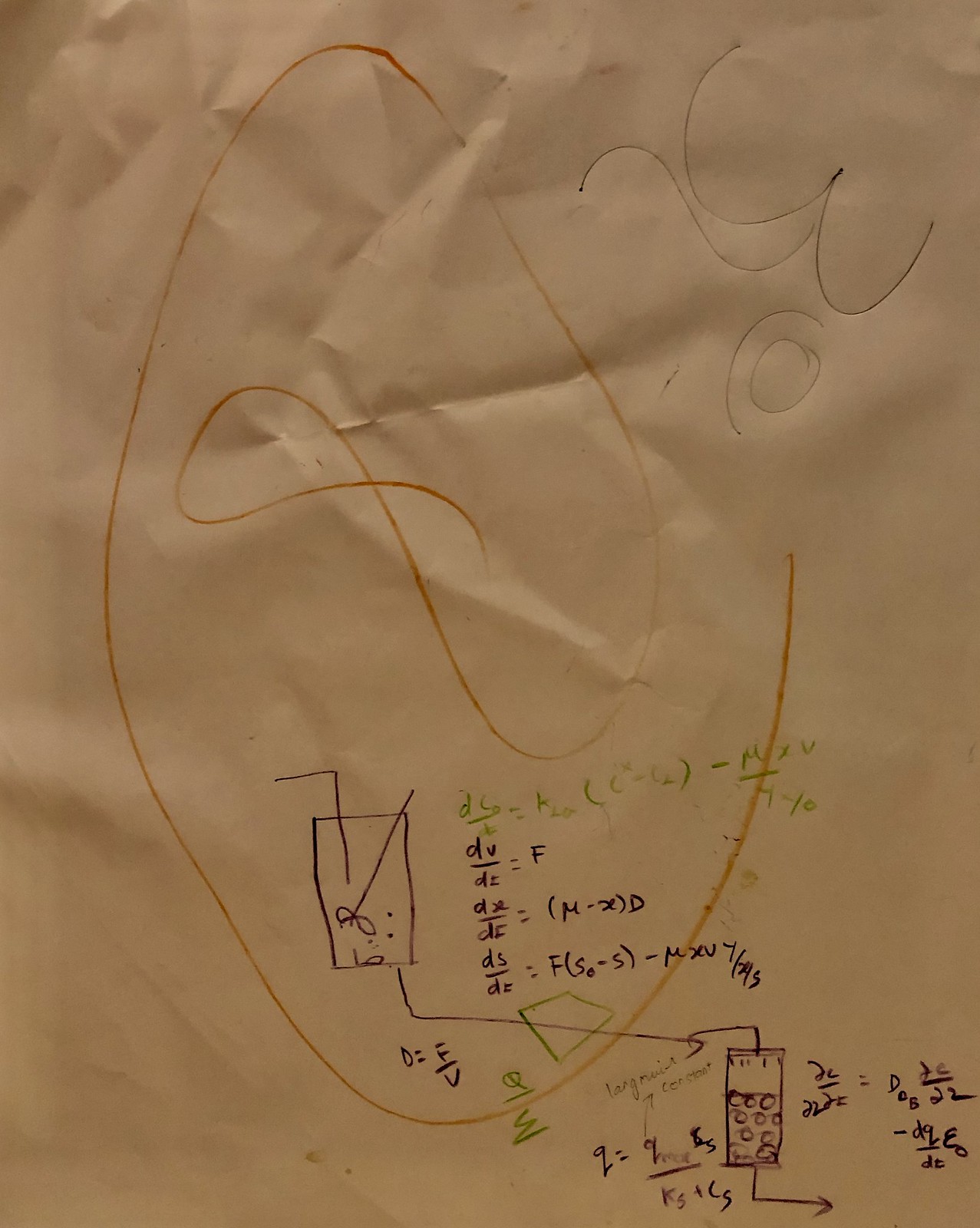A close-up photograph of a piece of paper, revealing only its central section. The paper is filled with various doodles and notes. Toward the top right, faint black biro squiggles can be seen, lightly etched into the paper. Dominating the height of the paper is a large swirl, drawn with either a brown pencil or a brown felt-tip pen. In the bottom area, an array of equations is visible. The first line of equations is inscribed in green pen, immediately followed by additional equations written more prominently in blue pen. Branching out from the equations, there is a complex diagram. Starting with a right-angled line that moves downward and then transitions into a tall rectangular shape before proceeding downward again, diagonal to the right. This geometric pathway continues into another tall rectangular shape filled with dots and concluded by another arrow moving downward and to the right.